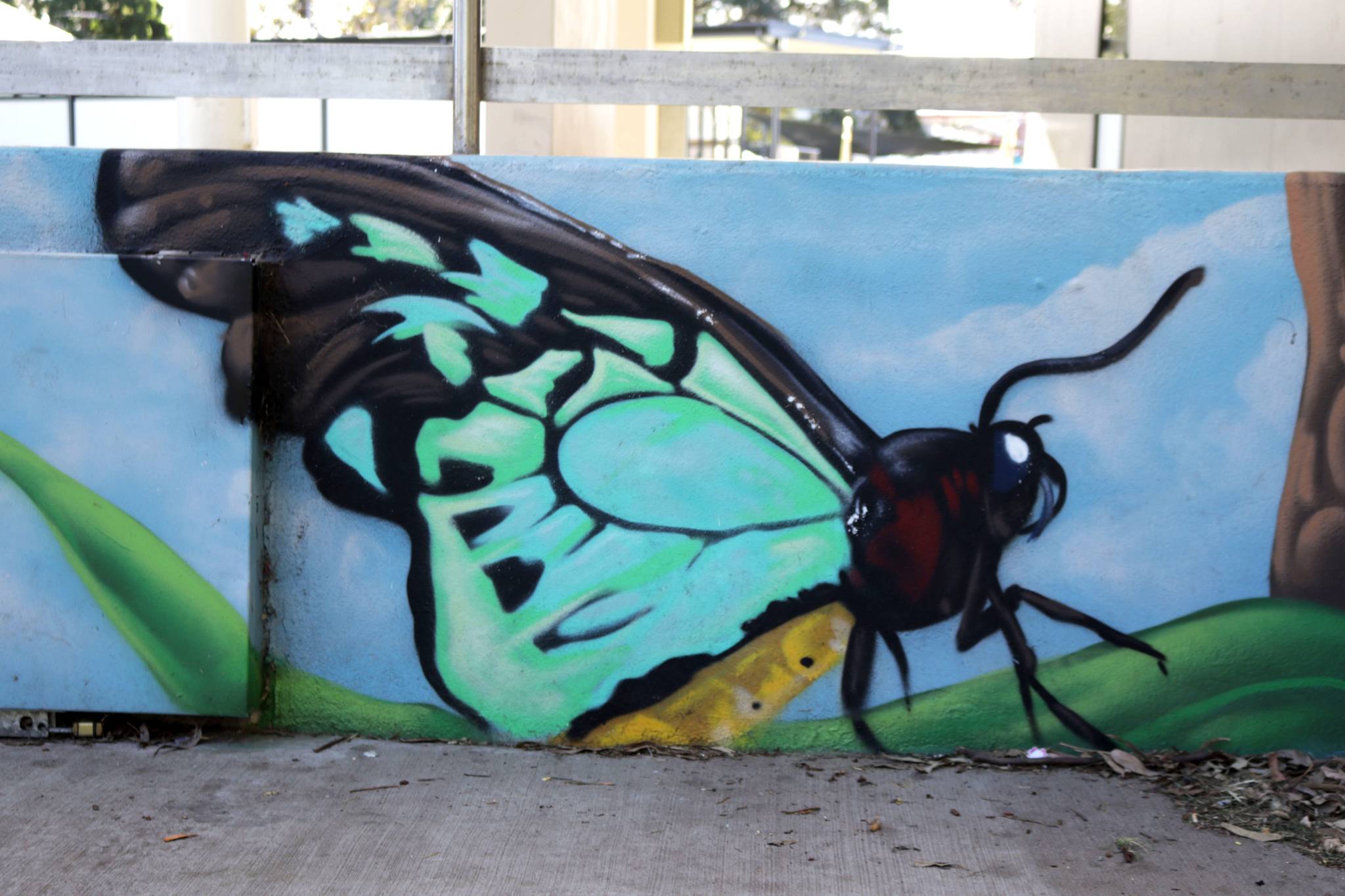This image vividly captures a mural painted on a low wall adjacent to a concrete walkway. The focal point of the artwork is a striking butterfly with a blend of teal, black, and green wings, and a golden yellow body. The creature's body also features areas of black and dark red, with prominent, beetle-like characteristics, including a large white eye and a single, noticeable antenna. The butterfly is perched atop a lush green leaf. To the right, part of a tree is visible, and the lower portion of the wall is adorned with an accumulation of fallen leaves. The background of the mural showcases a serene blue sky with scattered white clouds, creating a vivid contrast with the detailed insect. Beyond the wall, there is a suggestion of wooden railings, indicating that the walkway might lead up a ramp, enhancing the sense of depth and perspective in the scene.